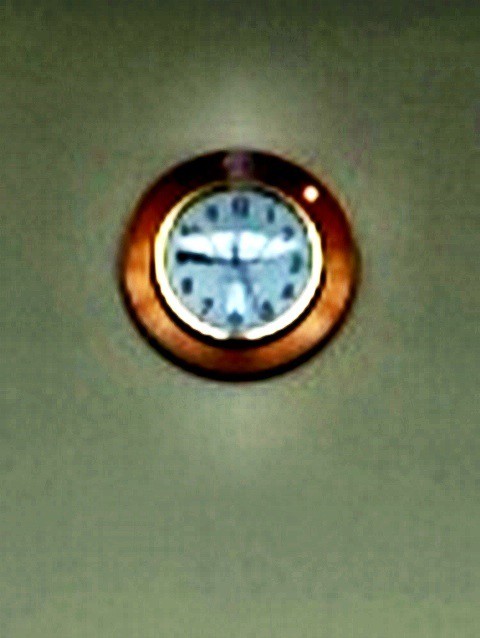In this detailed photograph of a wall-mounted clock, the sage green wall, darkening toward the top, provides a contrasting backdrop. The clock itself has a round design, featuring an outer edge that appears to be a brown wooden or copper metallic color. This peripheral frame is followed by a metallic ring and a reflective dot near the two o'clock position, indicating some form of polished surface. The face of the clock is white, with black numbers circling from 1 to 12. The black hands of the clock show the time at approximately 5:45, with the small hand just past the 5 and the long minute hand pointing at the 9. A faint reflection on the clock and slight out-of-focus elements suggest it may not be perfectly modern, adding a nostalgic or vintage charm to the image.